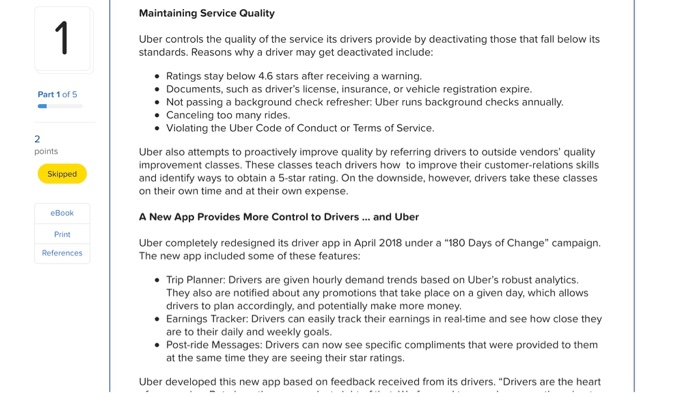**Detailed Caption:**

This image is a screenshot taken from an electronic device, displaying a section of text with a heading titled "Maintaining Service Quality." The text primarily discusses Uber's strategies for ensuring high service standards among its drivers. 

Uber maintains the quality of service by deactivating drivers who fall below its standards. Drivers may be deactivated for several reasons, including maintaining ratings below 4.6 after receiving a warning, failing to update essential documents such as their driver's license, insurance, and vehicle registration, and not passing annual background checks. Additional reasons for deactivation include canceling too many rides, and violating Uber's code of conduct and terms of service.

The text goes into further detail about Uber's proactive measures to improve service quality. One such measure is referring drivers to external vendors for quality improvement classes. However, these classes are to be taken by the drivers on their own time and at their own expense.

Towards the bottom of the screenshot, it discusses a new app designed to give more control to both drivers and Uber. This redesigned app was launched in April 2018 as part of Uber's "180 Days of Change" campaign. Key features of the new app include:
- **Trip Planner:** Provides hourly demand trends based on analytics.
- **Earnings Tracker:** Allows drivers to track their earnings in real-time and see how close they are to reaching their goals.
- **Post-Ride Messages:** Enables drivers to view specific compliments left by passengers.

The redesigned app was developed based on feedback from drivers, emphasizing their central role in Uber's operations. Unfortunately, the page cuts off, leaving the sentence "Drivers are the heart of..." incomplete.

On the left border of the screenshot, a large number "1" indicates that this is part one of five sections. Additional sidebar elements include "two points, skipped, e-book, print, and references." The background of the page is a nearly solid off-white color.